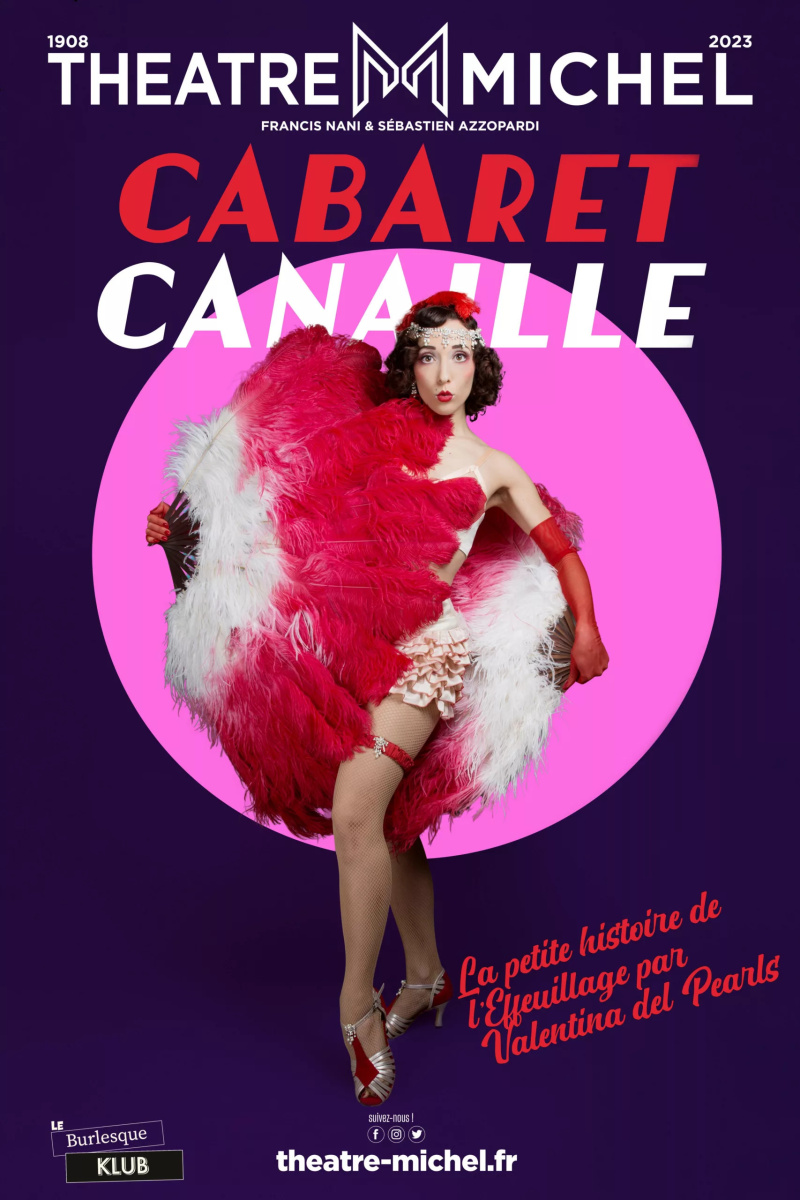This elegant poster advertises a captivating burlesque show at Theater Michel. Set against a dark blue background, the top of the poster features the text "Theater Michel" in bold white letters, flanked by "1908" on the left and "2023" on the right, paying homage to the theater's storied history. The show's title, "Cabaret Canaille," stands out prominently in bold red letters with "Canal" in white underneath. Central to the poster is a mesmerizing image of a cabaret dancer, characterized by her short dark hair, red lipstick, and stylish attire consisting of a small pink crop top, ruffled shorts, red garter, and red and silver high heels. The dancer holds large red and white feather fans in both her hands, one elegantly positioned in front and the other behind her, further accentuating her allure. She stands gracefully within a light pink circle that enhances her silhouette. Additional text in French appears at the bottom right in red, with specific details about the show: "La Petite Histoire de Le Voyage par Valentina de Pearls." At the bottom of the poster, the website "Theater-Michael.fr" is prominently displayed, inviting viewers to explore more about this enchanting burlesque experience.